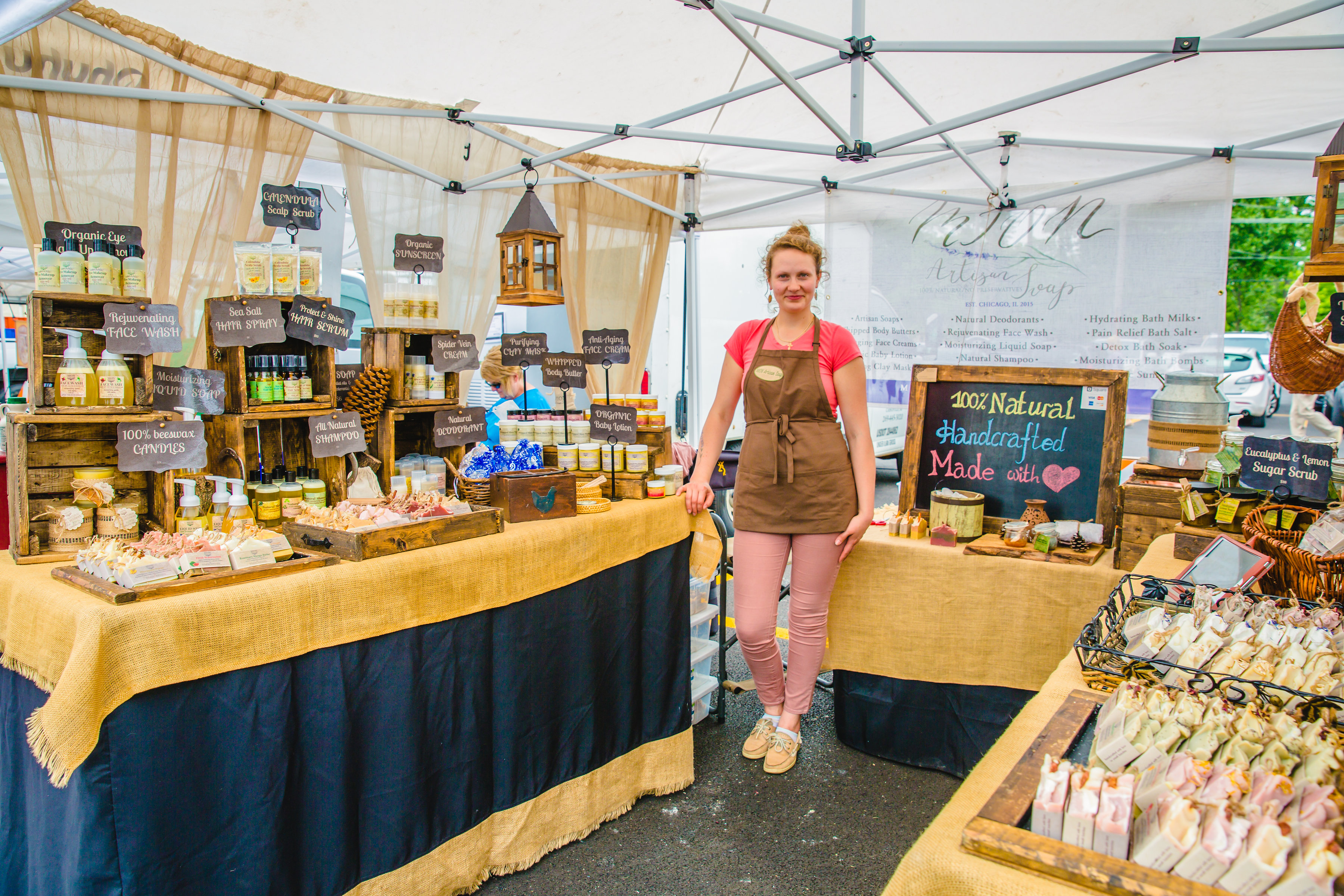The image depicts a woman, likely in her 30s, as the shop owner of a charming pop-up booth situated in a parking lot. The booth is set up under a white, semi-translucent tent, with visible parking lot lines and parked cars in the background, suggesting this may be a farmer's market or local business expo. The woman, who has auburn red hair tied in a bun and is wearing dangly earrings, is dressed in pink pants, a pink shirt, and moccasin slippers. Over her outfit, she wears a brown apron which bears a name tag or a logo that is not clearly readable.

She stands at the center of the booth, next to one of the three tables covered in cloths featuring striking gold and blue patterns. At each table, rustic-looking wooden boxes display various handcrafted beauty products such as organic body lotion, natural deodorant, all-natural shampoo, and organic sunscreen. These items are labeled with black signs and white text, enhancing their artisanal appeal. Among the signs, a central chalkboard prominently reads, "100% natural, handcrafted, made with heart." The booth also has a white, semi-transparent poster board displaying the business name in cursive, though it is somewhat hard to read. The overall setup is neat and inviting, with the woman posing with a gentle smile, reflecting the care and passion put into her craft.